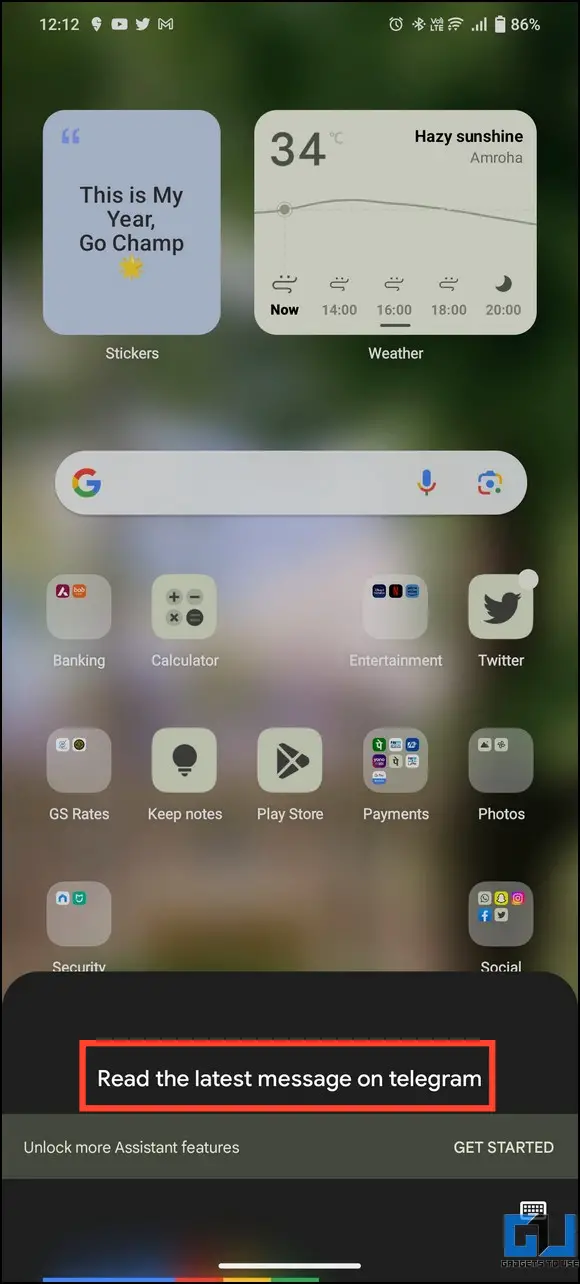This image is a screenshot from a smartphone's home screen. The background is a very blurry photo that is out of focus, displaying a blend of colors primarily featuring lavender and silver in the center. At the top, the colors transition to shades of green, culminating in very dark green at the very top.

Positioned on the left side of the screen in white font, the time is displayed as 12:12, without specifying AM or PM. On the right side, the battery icon is visible, indicating that the battery is charged at 86%. 

Below the time and battery icons, there is a lavender-colored square with rounded corners placed on the left side of the screen. This box contains the motivational text "This is my year, Go champ." To the right of this, there is a rectangular widget with a gray background and rounded corners. This widget is the weather forecast, displaying "34" (units not specified) on the left, with the description "Hazy Sunshine" on the right.

Central to the screen is the Google search box, a long rectangle with rounded corners. The Google 'G' logo is on the left side, followed by a small microphone icon and the Google Lens icon.

Below the Google search box, there are several folders for apps, all of which appear in gray. At the very bottom, a dark background hosts a white font text: "Read the latest message on Telegram." This text is enclosed in a red-lined rectangle.

The very bottom strip of the screen is gray, with white text that says "Unblock more system features" on the left side, and "Get started" on the right side.